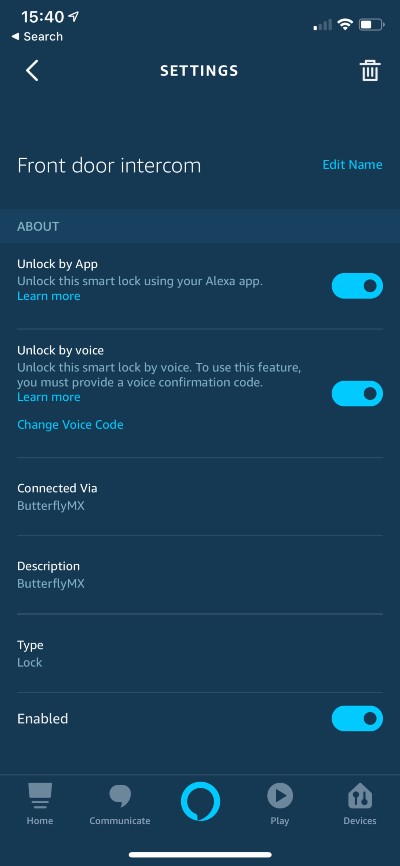This is a mobile screenshot of a settings page, featuring the phone's UI elements at the top: the clock on the left, and signal strength, Wi-Fi status, and battery life on the right. The settings header is prominently displayed at the top with a back arrow on the left. Below this, the device name "Front Door Intercom" is shown, along with an "Edit Name" option on the right.

In the first section, a blue bar labeled "About" is followed by descriptive text and interactive elements. The initial option, "Unlock by App," allows users to unlock this smart lock using the Alexa app. It includes a "Learn More" link and a dividing line for separation.

The next section labeled "Unlock by Voice" allows the smart lock to be unlocked via voice command. To use this feature, a voice confirmation code is needed. This section also contains a "Learn More" link and a "Change Code" link for further customization. The toggle buttons for these features are blue and pill-shaped with a dark blue circle indicating their current status.